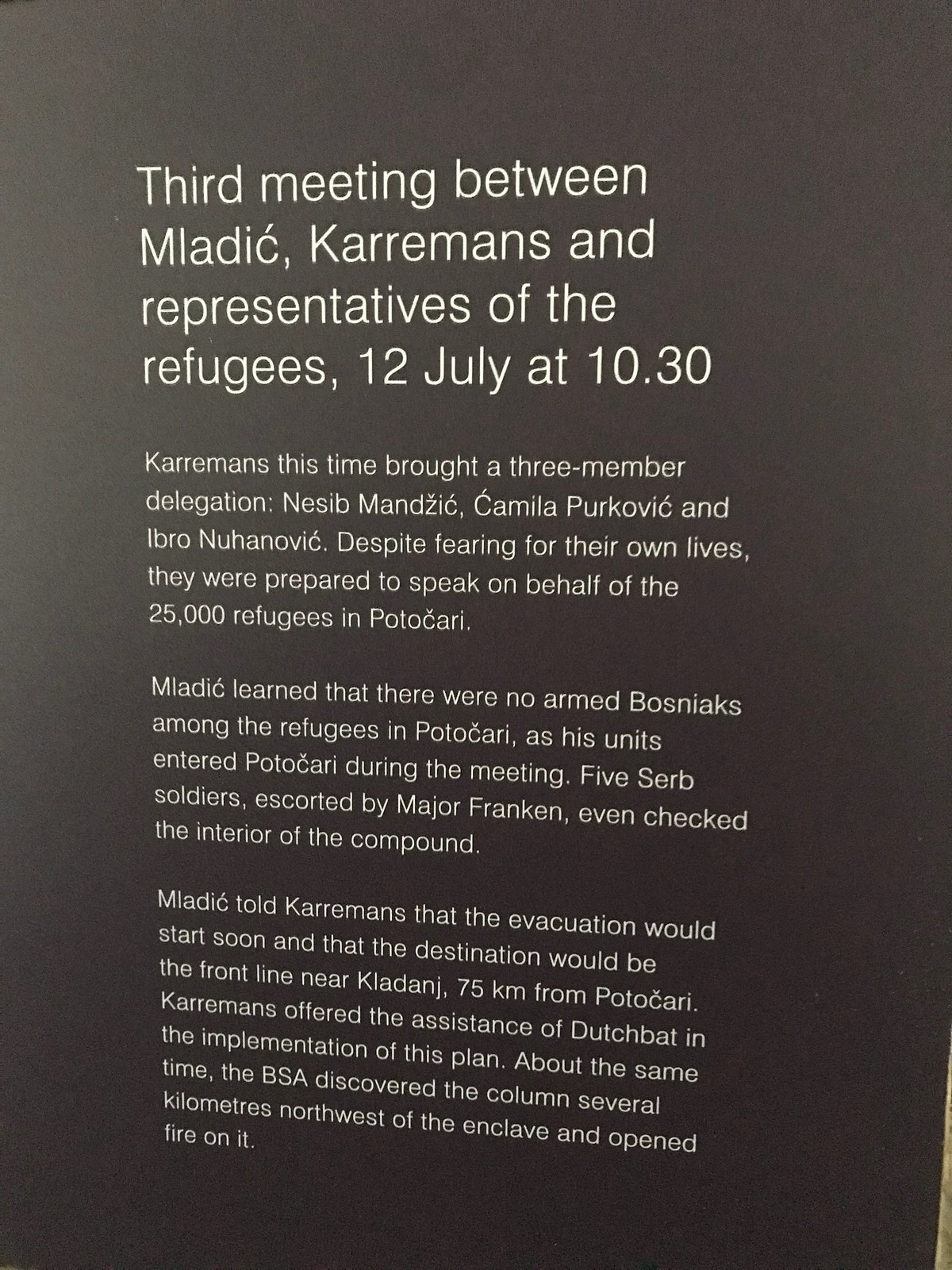The image features a dark, slightly washed-out black or dark brown sign with white or off-white text arranged in four distinct sections. The top section, with a larger font, reads: "Third meeting between Mladić, Karremans, and representatives of the refugees, 12 July at 10:30 AM." The subsequent paragraphs, in smaller font, detail that Karremans brought a three-member delegation comprising Nassib Manzik, Kamila Perkovic, and Ebro Nihonovic, who, despite fearing for their lives, were prepared to speak on behalf of 25,000 refugees in Potokhari. During the meeting, it was revealed that there were no armed Bosniaks among the refugees as Mladić's units entered Potokhari. Five Serb soldiers, escorted by Major Franken, checked the interior of the compound. Mladić informed Karremans that the evacuation would soon start, with the destination being the front line near Klenic, 75 kilometers from Potokhari, and that Dutchback assistance was offered for the plan’s implementation. Around the same time, the BSA discovered a column several kilometers northwest of the enclave and opened fire on it.